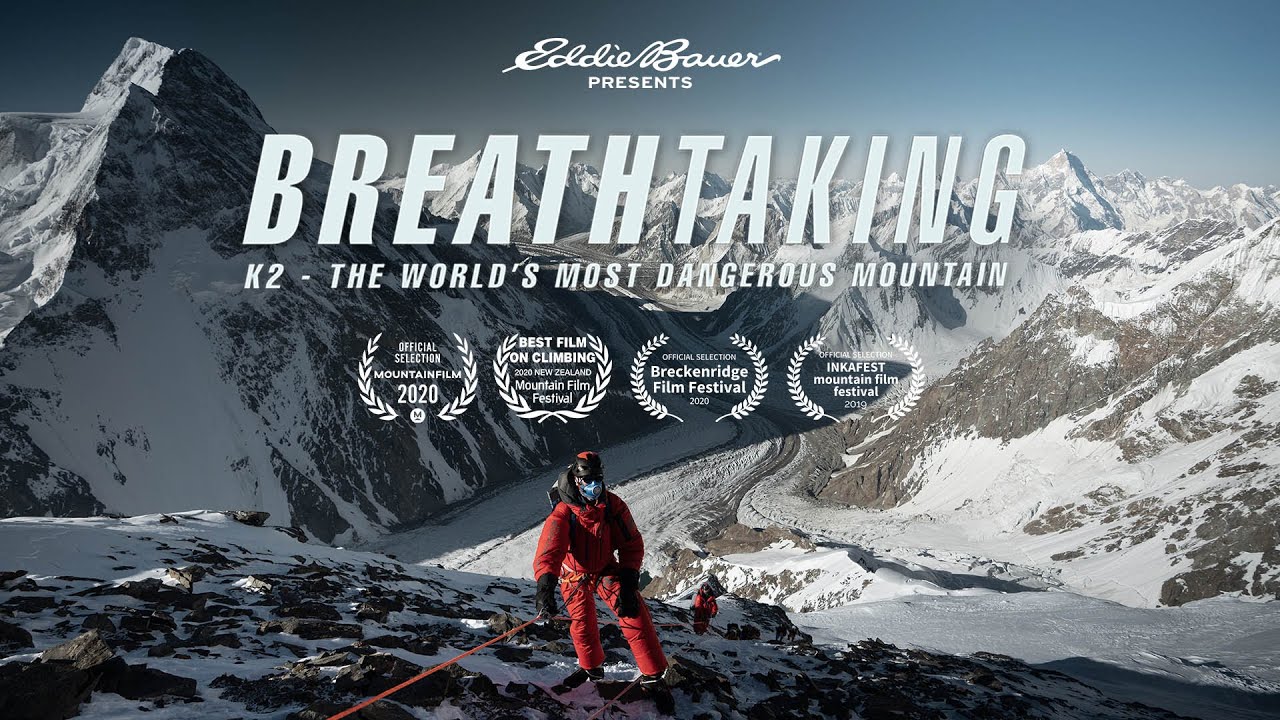In a stunning winter landscape, this advertisement for a film presented by Eddie Bauer showcases the breathtaking and perilous K2, renowned as the world's most dangerous mountain. Dominating the scene, large white text emblazons the message: "Eddie Bauer Presents Breathtaking K2, The World's Most Dangerous Mountain." This compelling image highlights the film's accolades, including "Best Film on Climbing" from the 2020 New Zealand Mountain Film Festival, and official selections at the Mountain Film 2020, Breckenridge Film Festival 2020, and Inca Fest Mountain Film Festival 2019.

Set against massive, snow-covered cliffs, the image captures the intense environment with two mountaineers clad in vivid red jumpsuits. The primary climber, distinguishable by his black backpack, mask, sunglasses, and hat, is navigating the hazardous terrain, while a second climber, also in red, can be seen beneath him. This gripping photograph not only emphasizes the dramatic and dangerous nature of K2 but also underscores the profound human spirit of adventure and endurance.